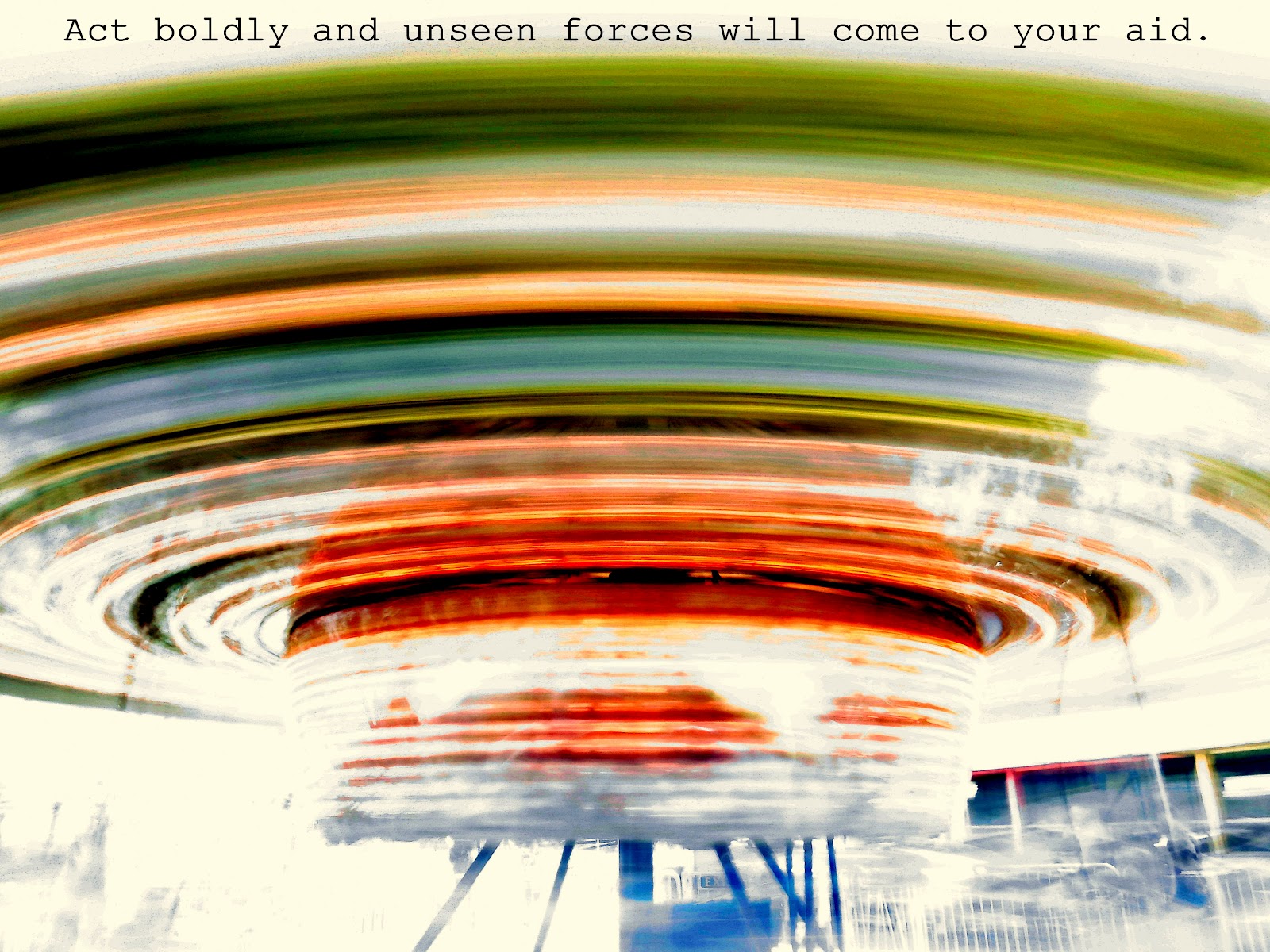The image captures the vibrant, swirling colors of a spinning ride at a carnival or fair, where the motion blurs the scenery, creating a dynamic and chaotic visual. In the foreground, you can see an array of vivid hues ranging from greens and blues to reds, whites, and pastels. The ride appears to be held aloft by blue posts or beams, with various cars or swings suspended by ropes or cables, though the riders themselves are not visible. The scene is set against a backdrop of distant building edges, roofs, gates, and entryways, adding layers to the composition. At the very top of the image, a message reads, "Act boldly and unseen forces will come to your aid," providing an enigmatic caption to this abstract yet captivating spectacle.